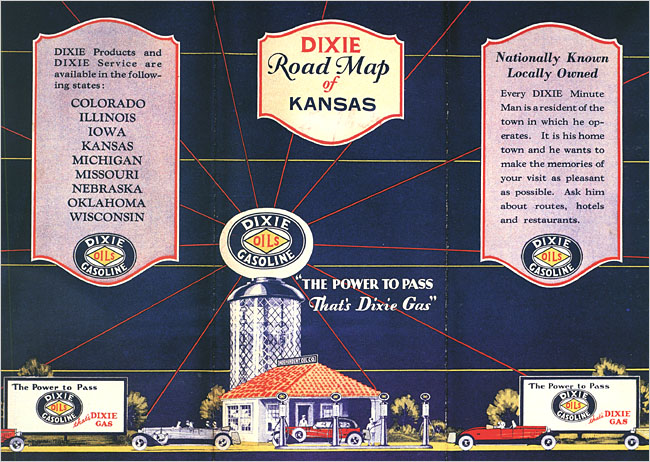The image is a photograph of an old, vintage illustration, possibly clipped from a magazine, depicting a detailed historical advertisement for Dixie Gasoline. Centered prominently is the "Dixie Roadmap of Kansas." The illustration features a green textured background with an intricate bubble map. In the middle, a large emblem showcases the text "Dixie Gasoline," with a rhombus containing the word "Oils" between "Dixie" and "Gasoline."

Above a detailed drawing of a Dixie gas station, there's a tall silver tower with an oval-shaped topper displaying the Dixie Gasoline logo—an oval within an oval with the primary text in dark blue. Radiating from this emblem are red lines, creating a sunburst effect.

To the left, the map lists states where Dixie products and services are available, including Colorado, Illinois, Iowa, Kansas, Michigan, Missouri, Nebraska, Oklahoma, and Wisconsin. To the right, the text declares "Nationally Known, Locally Owned," explaining that every Dixie Minuteman is a local resident dedicated to providing pleasant service and useful travel information about routes, hotels, and restaurants.

At the bottom, the motto "The Power to Pass as Dixie's Gas" reinforces the brand's appeal. The illustration's nostalgic aesthetic, complete with cars and historic buildings, adds to its charm as a piece of Americana and a testament to the storied legacy of Dixie Gasoline.